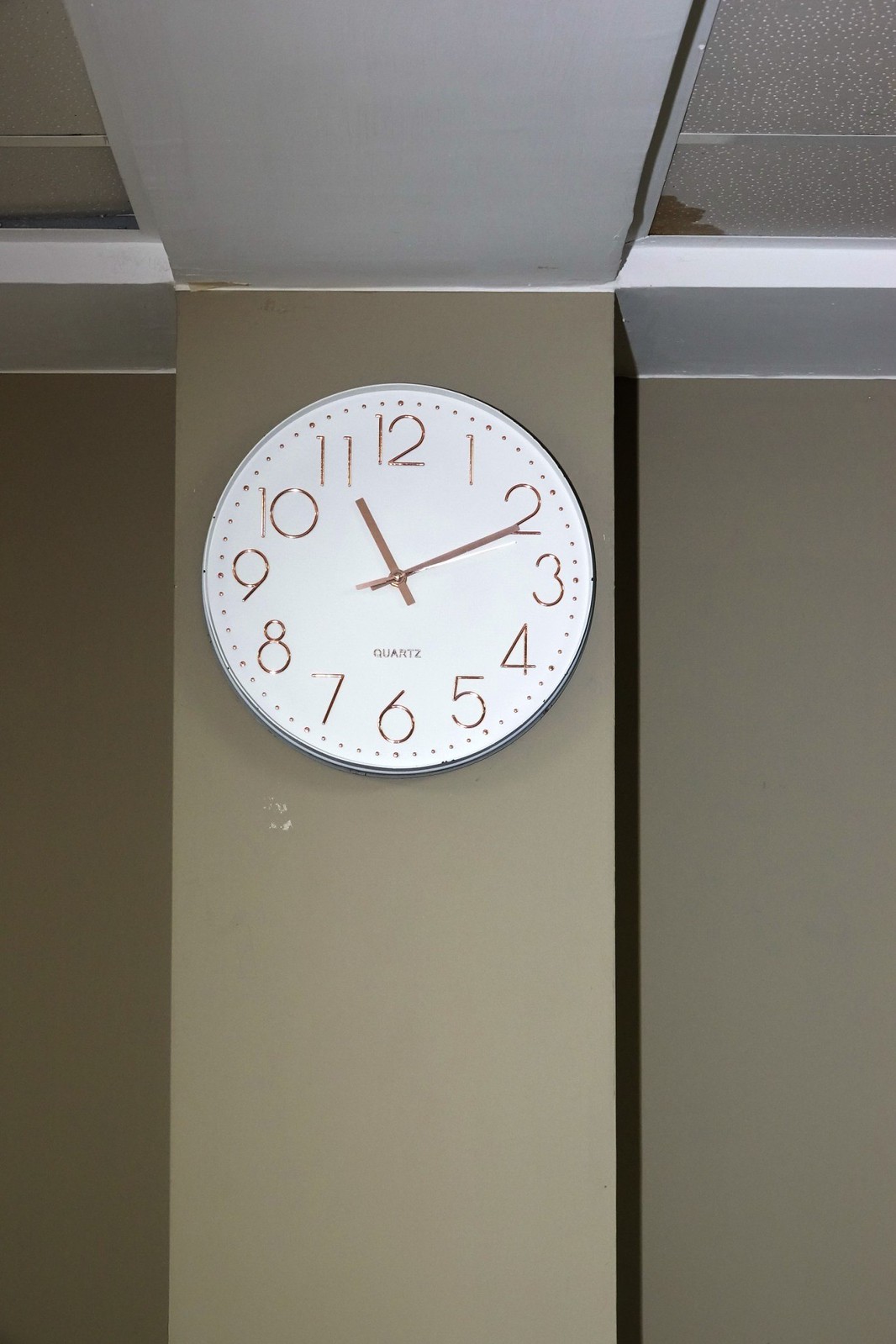In the image, the wall and background are predominantly gray, creating a muted, neutral backdrop. The ceiling, visible on both the left and right sides, is a pristine white, contrasting sharply with the gray walls. Centered in the frame is a clock with a traditional circular face, marked with brown numerals from 1 to 12. Surrounding these numerals are small dots that accentuate the edges of the clock face. The clock's minute hand points to the 2, and the hour hand points to the 11, both in matching brown. The hands are affixed with a small pin at the center of the clock. The ceiling tiles in the room are also visible and are of the perforated variety, adding texture and design to the otherwise plain ceiling.